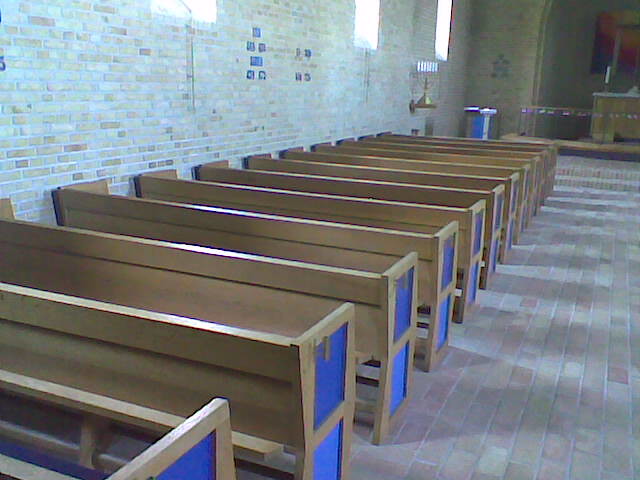This photograph captures an interior view of a traditionally decorated, likely older church, featuring a harmonious blend of brick, stone, and wooden elements. The image is taken from the central aisle, providing a clear perspective of the left side of the church. The foreground prominently displays a diagonal arrangement of around ten brown wooden pews extending from the bottom left corner to the upper right. Each pew features two distinctive dark blue rectangular inlays, bordered by the same brown wood.

The left wall of the church, running a little more than halfway across the image, is composed of muted red stone that appears whitewashed, adding an aged and serene ambiance to the scene. Embedded in this wall, there are three staggered windows: the lowest reveals just its bottom edge, the middle one shows about half of its structure, and the uppermost displays approximately three-quarters of its frame, all contributing soft natural light.

On the right side of the image, a brick-paved aisle leads the viewer's eye towards the altar area at the front of the church. Here, part of a brown wooden altarpiece is visible, featuring a single candle at one end. This altar, nestled within a slightly open space, possibly an archway, evokes a sense of sacredness and focus within the religious setting.

Overall, this image depicts the intimate, contemplative atmosphere of a historical church interior, characterized by its detailed wooden pews, rustic stone walls, and softly illuminated windows.